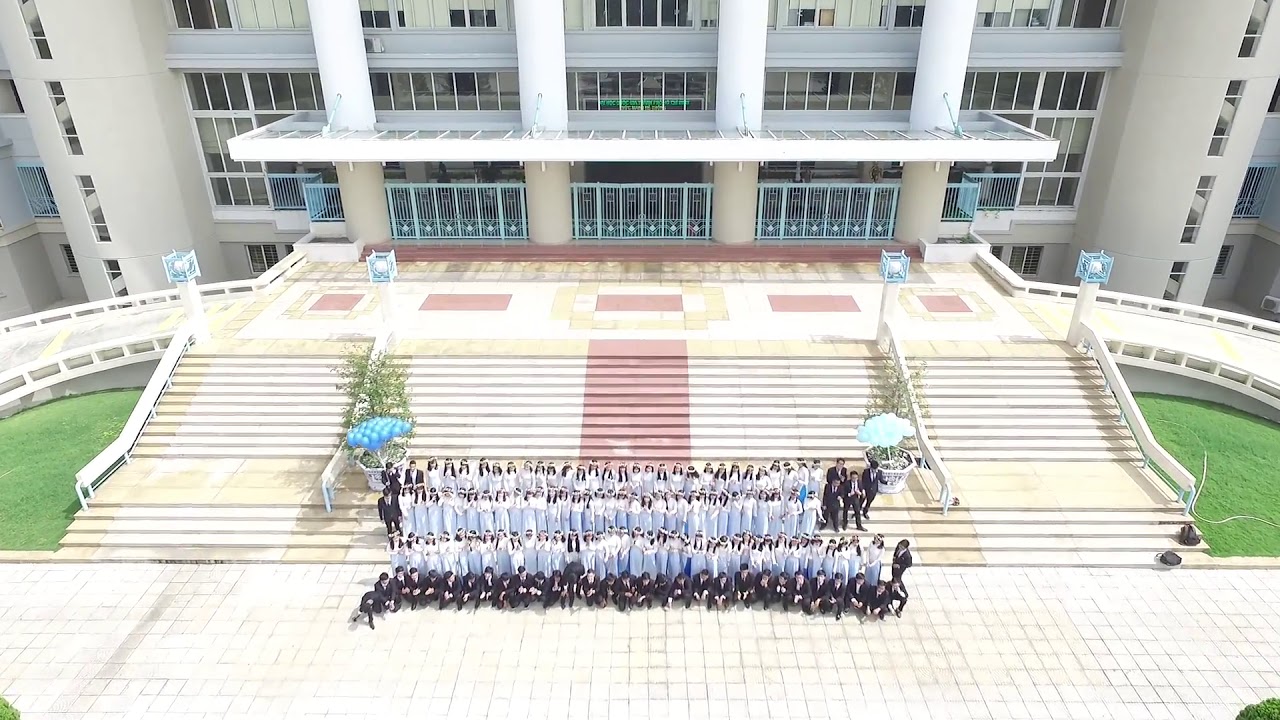This landscape-oriented color photograph, captured from high above using a drone, features a large group of graduating students arranged in three rows. The students, all wearing white robes, stand in front of a grand staircase leading up to an imposing multi-story building, which could be a university, characterized by its numerous windows and white columns. The front row, consisting of students in black, is kneeling. The background reveals a meticulously clean edifice adorned with blue and white metal gates, interspersed with red marble insets and a red stripe at the center of the stairway. Checkered ground patterns extend in front of the steps, flanked by greenery on both sides. Despite being unable to discern individual facial features due to the high vantage point, the image captures the stark contrast of dark hair among the students, highlighting a sense of uniformity and regality in this significant event. Blue balloons in pots add a celebratory touch, while the overall composition underscores a moment of formal occasion and collective achievement.